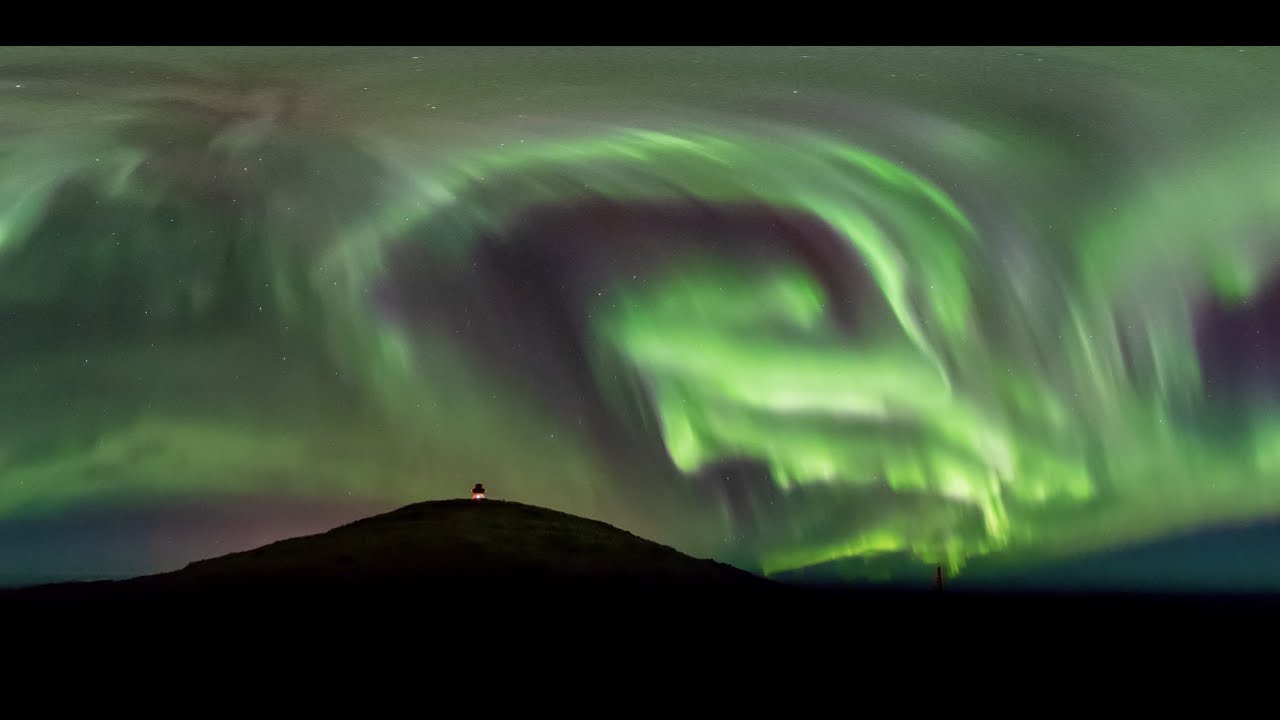The image captures the mesmerizing Aurora Borealis lighting up the night sky. A person, silhouetted and possibly sitting on a hill or a mountaintop, gazes at the breathtaking display. The landscape is cloaked in darkness, turning the hill into a mere silhouette against the vibrant sky. The Aurora Borealis showcases an incredible mix of colors, including vivid greens, purples, blues, and perhaps a hint of pink, forming erratic, swirling, and wavy patterns. The ethereal lights contrast beautifully against a backdrop that ranges from purplish-blue near the horizon to deeper shades of green and black higher up. Stars can be faintly seen peering through the celestial display, adding to the enchanting atmosphere.